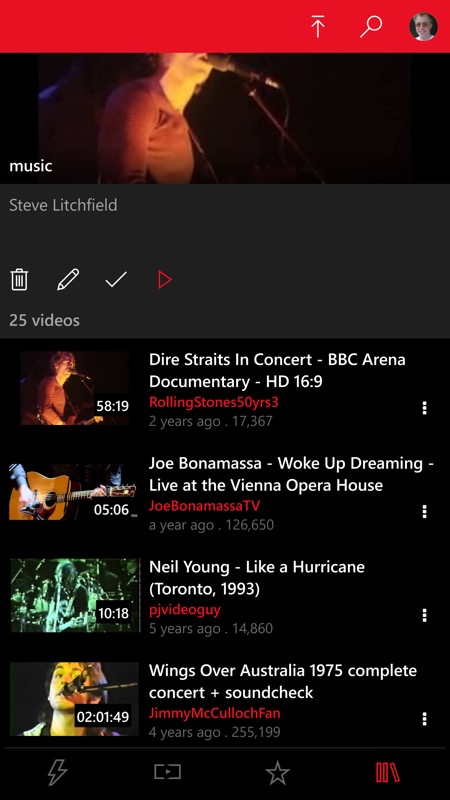A screen capture showcases a browsing window for streaming music content, distinguished by a red border at the top featuring navigational icons—including a forward button, a magnifying glass, and a profile picture. Beneath the red border, a header labeled "Music" appears, followed by a gray box displaying the name "Steve Litchfield." In the gray box, there are icons for a trash can, pencil, a check mark, and a red triangle, as well as text stating "25 videos."

Below this section, four thumbnails are displayed, each representing a different music video. The first thumbnail highlights a "Dire Straits Concert, BBC Arena Documentary" in HD with a 16:9 aspect ratio. It carries tags indicating it was uploaded 2 years ago and has accrued 17,367 views.

The second thumbnail features "Joe Bonamassa, Woke Up Dreaming, Live at the Vienna Opera House" from John Bonamassa TV. This video, uploaded a year ago, has garnered 126,650 views.

The third thumbnail presents a clip of "Neil Young, Like a Hurricane, Toronto 1993" from PJ Video Guy. This video was posted 5 years ago and has 14,860 views.

Finally, the fourth and last thumbnail in this row is of "Rolling Stone, 50 Years", uploaded 3 years ago.

Overall, the screen capture provides a detailed interface for Steve Litchfield's music video collection, displaying a range of concert footage and music documentaries from various artists.